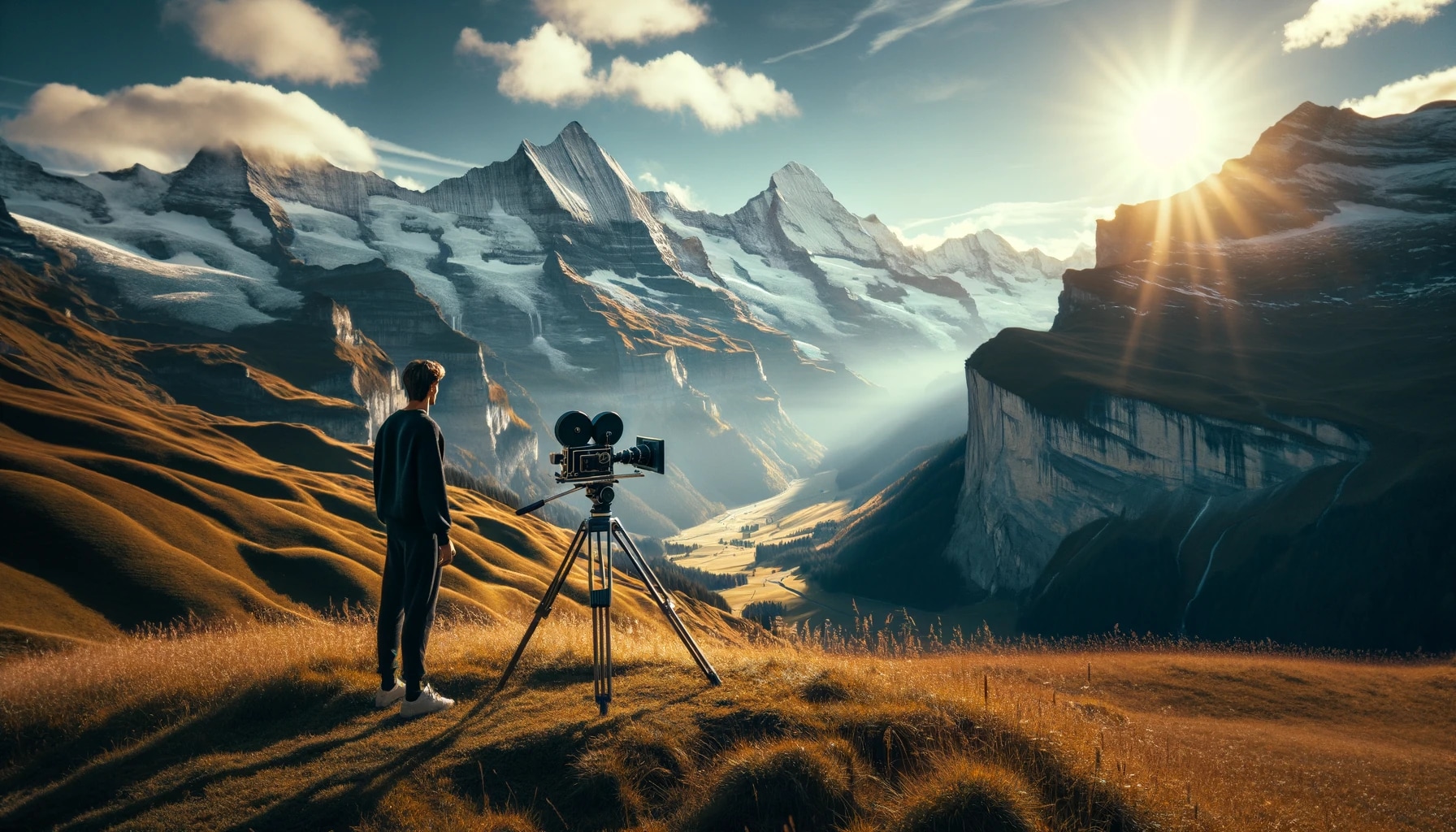This detailed painting captures an outdoor scene in a mountainous landscape at sunrise. A young white man with brown hair, dressed in what appears to be a gray shirt and pants, stands in the lower left-hand corner behind a tripod-mounted film camera. His blue sneakers are visible, and he gazes intently at a majestic view. The foreground features grassy soil and a large rock, adding depth to the image, while the midground consists of rolling hills that lead the eye towards a background of majestic, snow-capped mountains. The blue sky is dotted with white clouds, and the sun, its bright white rays tinged with yellow, rises spectacularly from behind a mountain in the upper right-hand corner. Despite its vivid and detailed execution, there is a surreal quality to the painting, making it hard to distinguish if it is a real landscape or an imaginative creation.